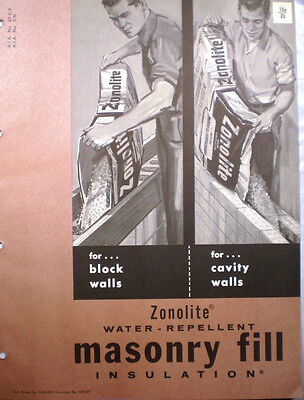This is a vintage advertisement from the 1950s for Zonolite Water Repellent Masonry Fill Insulation, featuring black and white illustrations on a brownish-orange background. The ad is in portrait orientation, and appears to be a photograph of the original poster, showing staple marks on the left side. The main image, located on the right half of the ad, is divided into two sections. On the left, a man is depicted pouring insulation into a wooden canal, labeled "for block walls," while on the right, he is seen filling between a brick wall, labeled "for cavity walls." Below these images, the product name "Zonolite Water Repellent Masonry Fill Insulation" is prominently displayed in black letters.